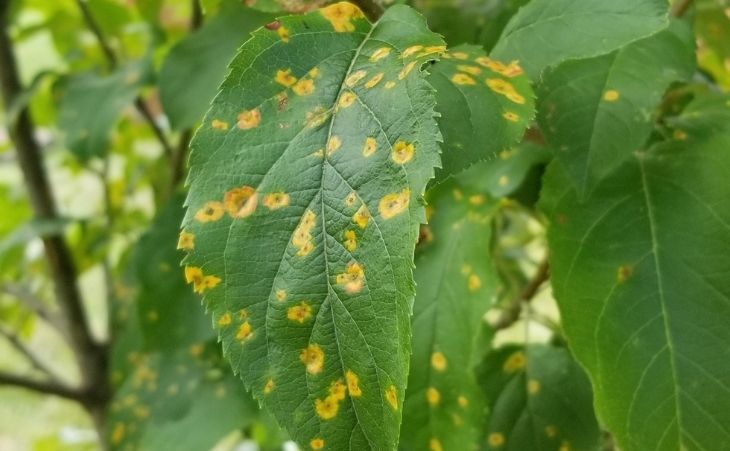This is a real-life, close-up photograph taken in landscape orientation during the daytime. It focuses on a green leaf that is prominently centered in the frame. The leaf is heavily dotted with unsymmetrical, circular yellow spots, each with a brown center, suggesting it is afflicted by a disease. Behind this main leaf, the background is blurred, revealing other leaves from the same plant, some of which also display similar yellow and brown spots indicating disease, while others show fewer signs of affliction. Among these leaves, thicker brown branches can be seen, suggesting the plant may be some type of tree. The context around the leaf hints at a bushy green space in a natural setting.